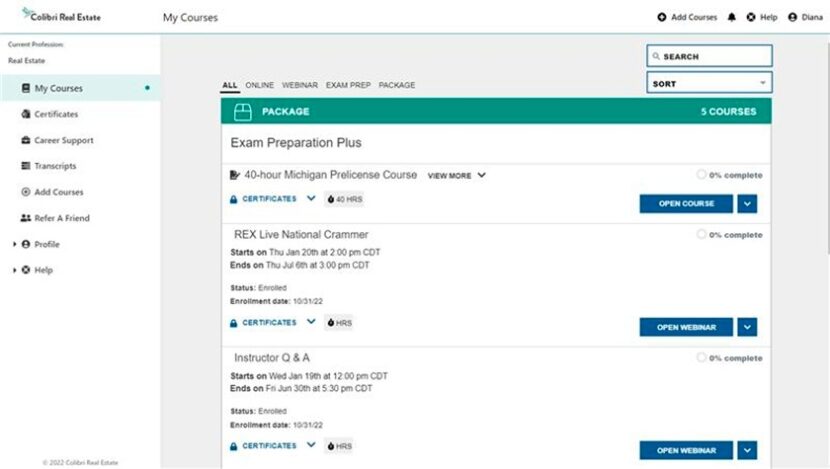Detailed Caption: 

The screenshot depicts a detailed class schedule page from an online real estate course platform. The page has a clean, white background and at the very top in bold, prominent letters is the title "Real Estate - My Courses." On the right-hand side of the header, there are options to add courses, access health information, and view the user's profile.

Just below the header, a horizontal blue line separates the header from the main content. The page is then divided into two sections. On the left is a vertical navigation bar, which includes options such as My Courses, Certificates, Career Support, Transcripts, Bad Courses, Refer a Friend, Profile, and Health. The navigation bar has a highlighting feature that illuminates the current selection or the option over which the cursor hovers.

To the right of this navigation bar lies a gray-interfaced section. This area contains two white boxes surrounded by blue outlines, labeled "Search" and "Sort." Below this section, a prominent green bar with white text states "Package: 5 Courses." Underneath this, there is a label for "Exam Preparation," which lists three specific classes within this category: Q&A, Understanding, and Certificates. Each class entry can be expanded to read detailed descriptions and additional information about what each course entails.